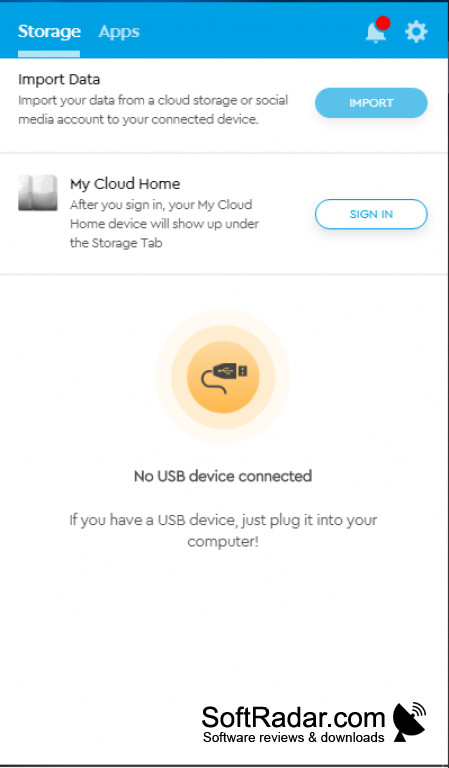This is an image of a website with a clean and user-friendly interface. The top of the website features a blue header displaying the words "Storage" and "Apps," with "Storage" being underlined. To the right of these words, there is an alert bell icon adorned with a red notification circle. Nearby, there is an icon of gears symbolizing the settings menu.

Below the header is a white section introducing the "Import Data" feature. The text reads: "Import your data from a cloud storage or social media account to your connected device." A blue "Import" button offers immediate action. This section is divided by a light gray line.

Further down, the section titled "My Cloud Home" appears. To the left is a black and white box. Text explains, "After you sign in, your My Cloud Home device will show up under the Storage tab." This section includes a blue-outlined, white button labeled "Sign In" in blue text.

Below, there is a yellow circular section with a visualization that appears to be a cable connecting to a port. The port and cable are depicted in black, transitioning to lighter yellow and pinkish hues. Accompanying text states, "No USB device connected. If you have a USB device, just plug it into your computer."

At the bottom of the webpage, "softradar.com" provides soft reviews and downloads, complete with an image of a radar.